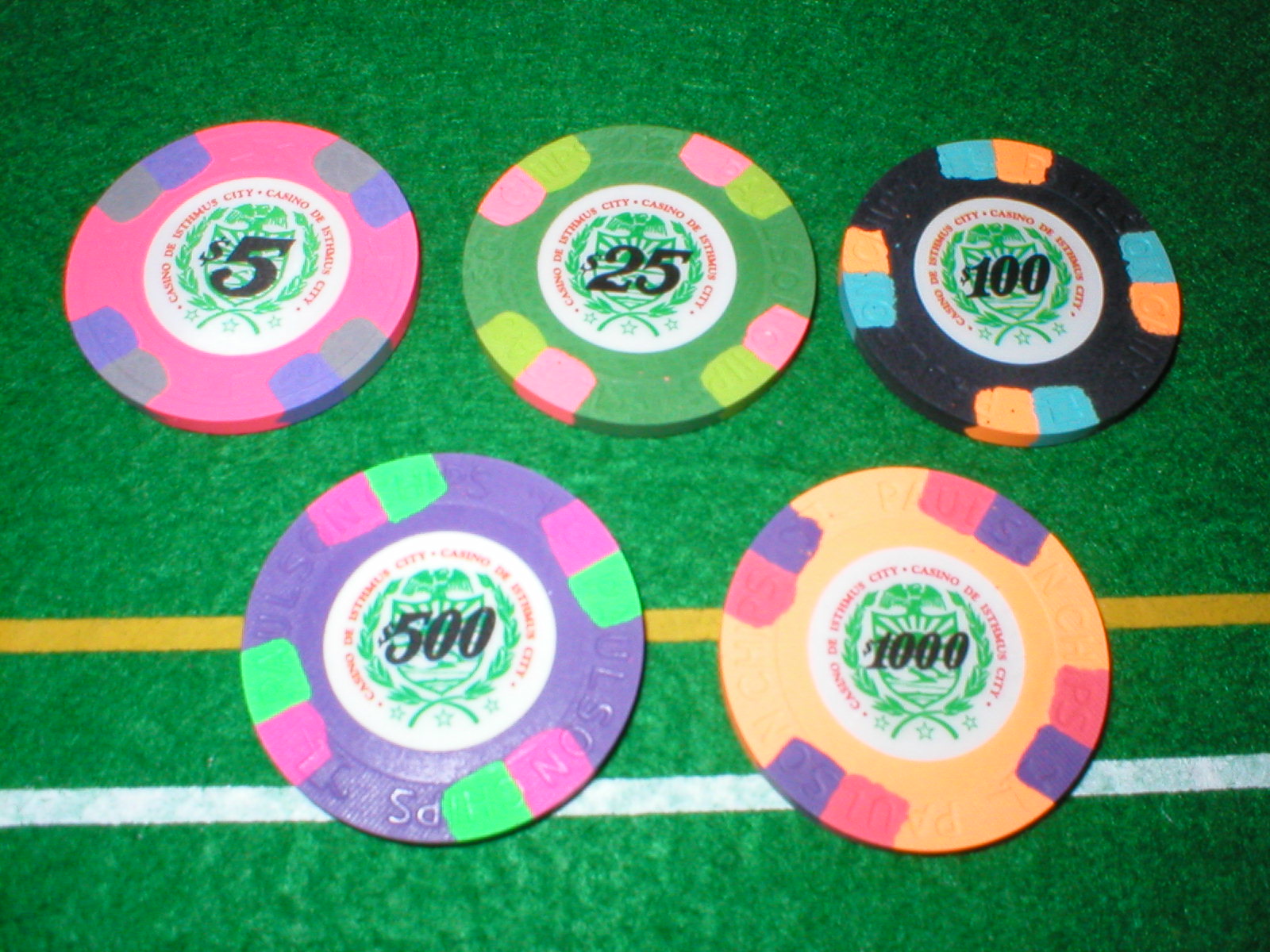A detailed color photograph taken at a casino features five vividly colored poker chips laid on a green felt poker table with two horizontal lines, one yellow and one white, in the background. The poker chips are arranged with three at the top and two at the bottom. The top left chip is pink, purple, and gray, marked with the number five, indicating a $5 value. Next to it is a green, pink, and lighter green chip marked with $25. The top right chip is black with orange and blue, marked with $100. On the bottom left is a purple chip with pink and mint green accents, marked with $500. The bottom right chip is peach with purple and pink, marked with $1,000. Surrounding the monetary values on each chip are the words "Casino" and a partially legible city name, indicating these tokens are from a specific casino.